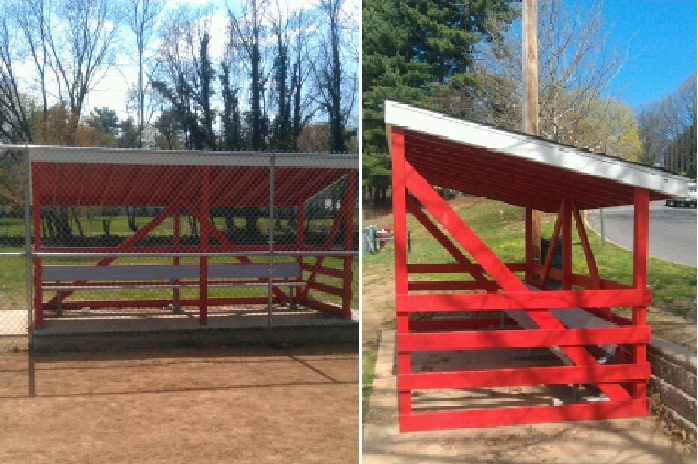The image is a composite of two vertical, rectangular photos of a baseball dugout, taken from different angles, positioned side-by-side. The dugout, situated in a park and located near a street, features distinct red and white wooden planks forming an enclosure. The front view, seen on the left, shows a dugout set behind a silver chain-link fence, with a white bench inside and brown dirt in front. The structure has horizontal wooden planks, with some vertical ones for support, and is topped by a sloped roof painted white on the trim and red underneath. Trees, some with leaves and some bare, are visible behind it, along with a glimpse of the bright blue, cloudless sky. The side view, depicted on the right, highlights the vertical and horizontal wooden planks and reveals more details of the white fascia of the roof. This angle also shows a large wooden pole and additional trees with the clear sky dominating the top right. A road is visible in the background with a vehicle traveling down it.